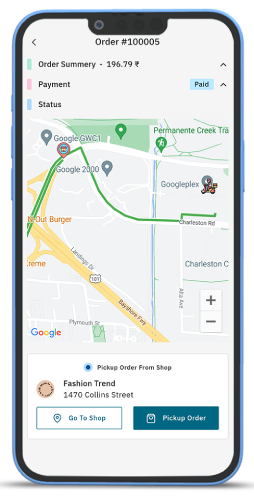The image depicts a smartphone screen displaying the interface of an order tracking application.

At the top of the screen, there is a black back arrow. Centrally positioned at the top is the text "Order Number 100005". Below this, a green square labeled "Order Summary 19679" features an upward arrow. 

The next section is titled "Payment" with a pink square to the right, indicating "Paid" in blue text, accompanied by another upward arrow. The "Status" section follows, marked in blue.

The screen prominently showcases a map below these sections. Additionally, there is a highlighted button featuring a dot, labeled "Pick Up Order from Shop". Adjacent to this button, the text "Fashion Trend, 1470 Collins Street" is visible. Beneath this, in white text with blue lettering, the option "Go to Shop" is provided.

To the right side of the screen, a blue square icon with a shopping bag and white text inside states "Pick Up Order". The map itself displays various areas marked in yellow and green, outlining the route to the store for collection.